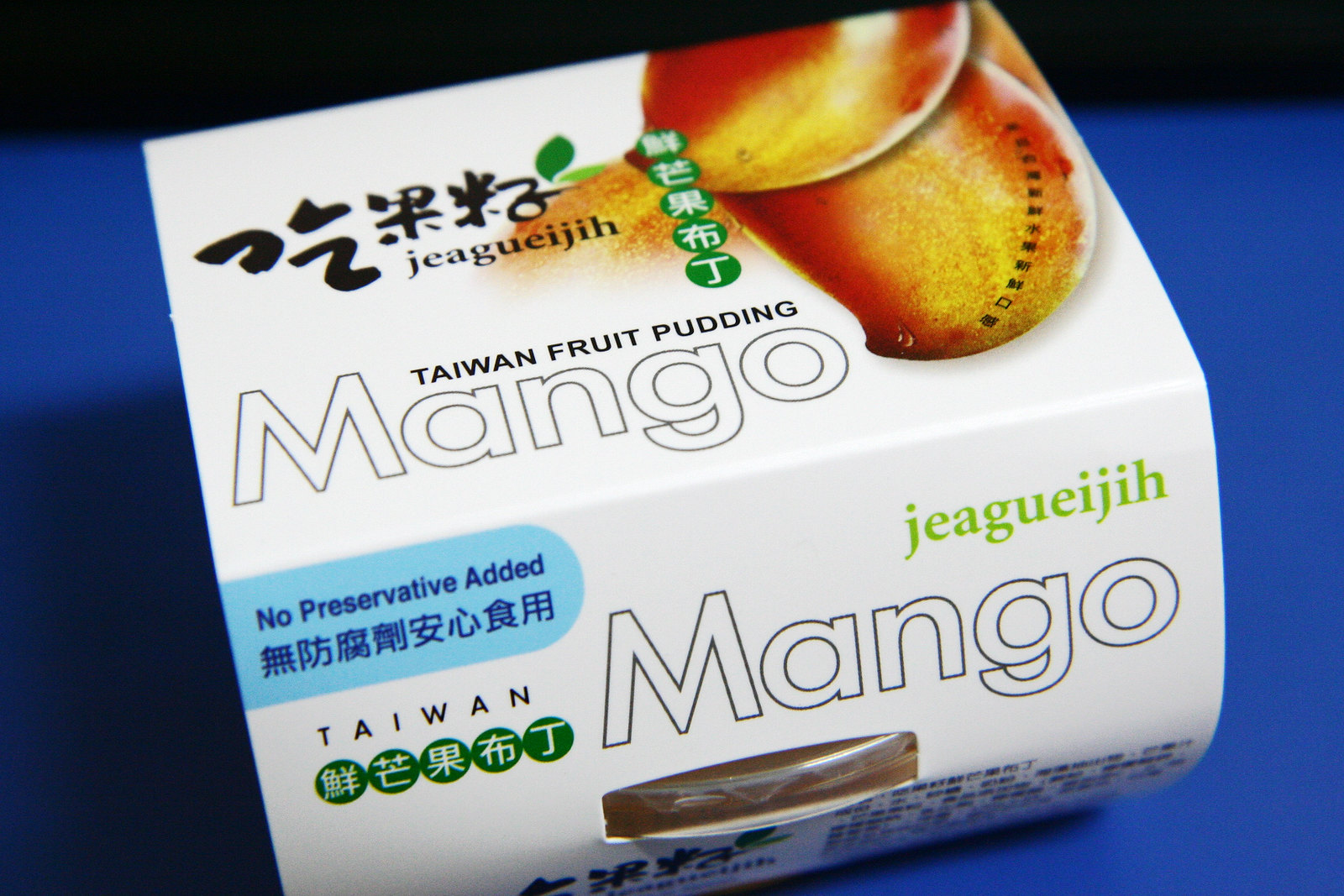This captivating image, formatted as a horizontal rectangular poster, showcases a vibrant mango product packaged in a white cardboard container. The container prominently features a reddish-orange and yellow mango image. At the top of the package, bold white letters with a dark outline spell "Mango,” and above that, black text reads "Taiwan Fruit Pudding." To the left of the container’s top, there are some Asian characters. The front of the packaging also includes a blue label stating "No Preservative Added" both in English and in Asian script below. Additionally, the product highlights the name "J-E-A-G-U-E-I-J-I-H," adorned in green, accompanied by a detailed image of a cup filled with a brown liquid, partially visible through the container. The entire product rests against a striking blue background, enhancing the colors and the text of the packaging.